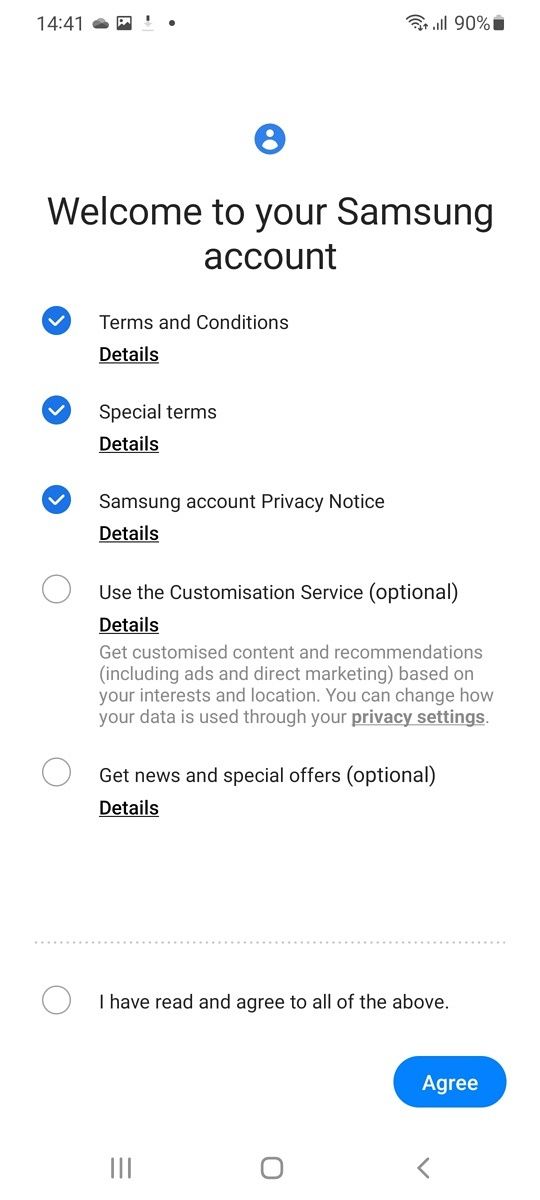The image displays the front screen of a smartphone, likely a Samsung model, showing the "Welcome to your Samsung account" page. The time is displayed in the upper-left corner as 14:41, accompanied by a partly cloudy weather icon. The top-right corner shows icons indicating full Wi-Fi and cell phone connectivity along with a battery level at 90%.

The main focus of the screen is the Samsung account welcome interface. At the top, a blue circle contains a stylized white figure representing a person. Below this, the text "Welcome to your Samsung account" is prominently displayed. 

Below this welcome message, there are several terms and agreements sections, each with corresponding blue checkboxes that are checked:
1. **Terms and Conditions** (Details underlined)
2. **Special Terms** (Details underlined)
3. **Samsung account privacy notice** (Details underlined)

There is also an optional section titled "Use the customization service" with an unchecked white box. This section offers to provide customized content and recommendations, including ads and direct marketing based on the user's interests and location, with instructions on how to modify data usage through privacy settings.

Another optional section titled "Get new and special offers" includes an unchecked box, indicating consent for receiving news and special offers.

The interface continues with some white space followed by a line of dots, underneath which a statement reads, "I have read and agreed to all the above," along with an empty checkbox. At the very bottom, a prominent blue button labeled "Agree" in white font invites the user to give their consent.

Finally, at the bottom of the screen are three navigation symbols: three vertically aligned dots, three horizontal dashes, a small box, and a left arrow, likely for menu navigation and return options. This detailed interface shows the initial setup and consent process for a new Samsung account on a mobile device.